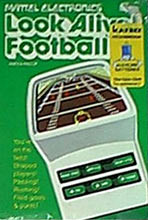The photo showcases a vintage electronic football game set against a green advertisement background. The advertisement prominently displays the text "My Little Electronics Look Alive Football." In the bottom left corner, there is a yellow sticker with unreadable text. Additional illegible writing appears on a small white rectangular shape, which flares out at the top before tapering and has a flat upper edge.

The electronic game itself features six green buttons along the lower edge. At the top of the device is a small screen displaying a brown track, segmented into white rectangles. The sides of the track are marked with lines, with an orange marker on the right of one of the rectangles and two orange markers on the upper left rectangle. Towards the bottom of the screen, there is a small yellow icon resembling a head.